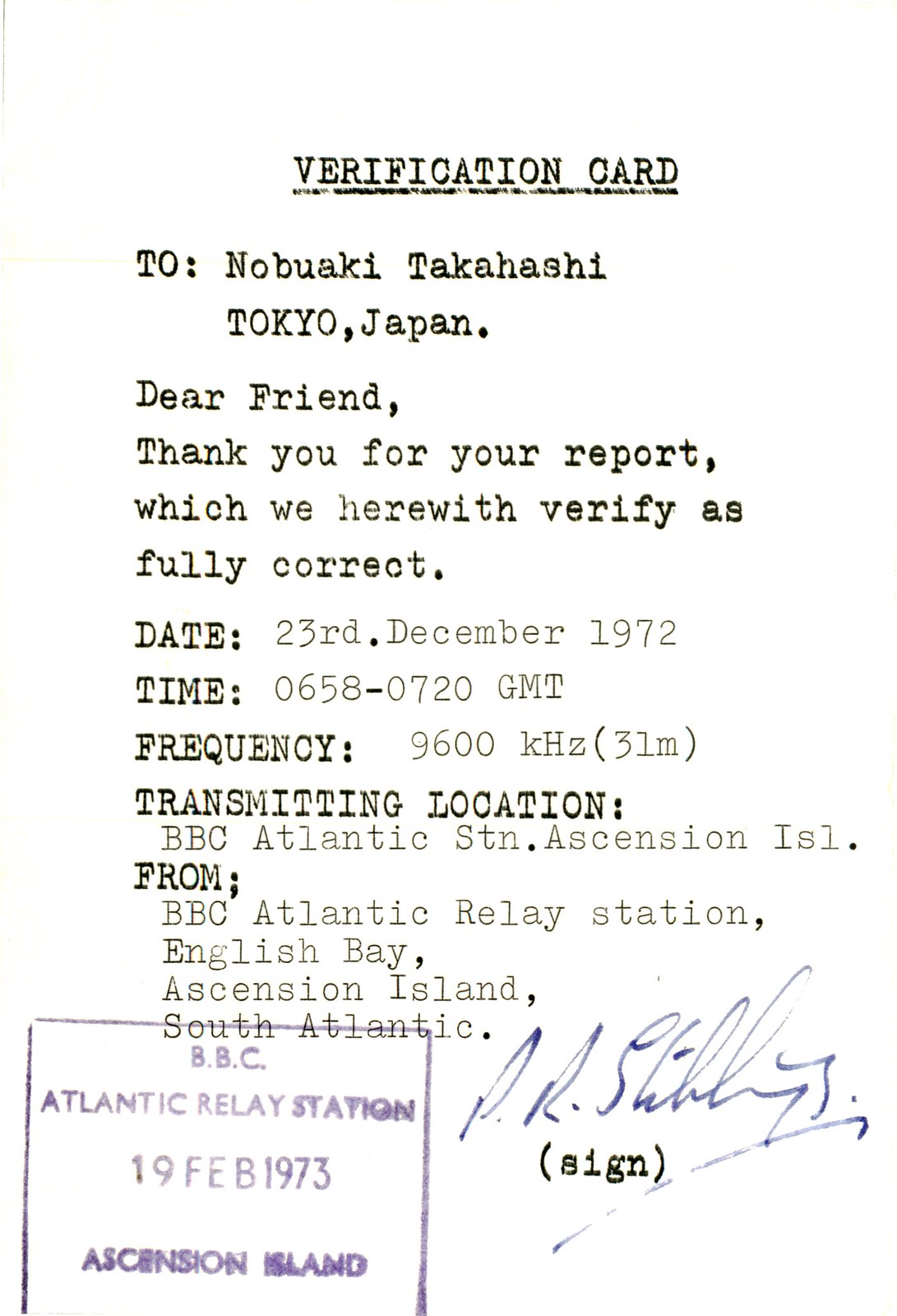This image shows a verification card, typewritten with black ink on a pristine white background, exhibiting the distinct, uneven alignment of a classic typewriter. The card is addressed to Nobiyuki Takahashi in Tokyo, Japan. At the top, it reads "Verification Card" underlined, followed by "To: Nobiyuki Takahashi, Tokyo, Japan." Below, it says, "Dear friend, thank you for your report, which we herewith verify is fully correct." The card includes specific details: Date: 23rd December 1972; Time: 0358-0720 GMT; Frequency: 9600 kHz, 31M; Transmitting Location: BBC Atlantic Station, Ascension Island; and From: BBC Atlantic Relay Station, English Bay, Ascension Island, South Atlantic.

In the lower left corner, there's a purple stamp that reads "BBC Atlantic Relay Station, 19th February 1973, Ascension Island," signifying the authenticity of the document. Adding a personal touch, the lower right corner features a handwritten signature in blue ink, with the annotation "(signed)" beneath it. The card's orderly yet nostalgic presentation highlights its historical significance.